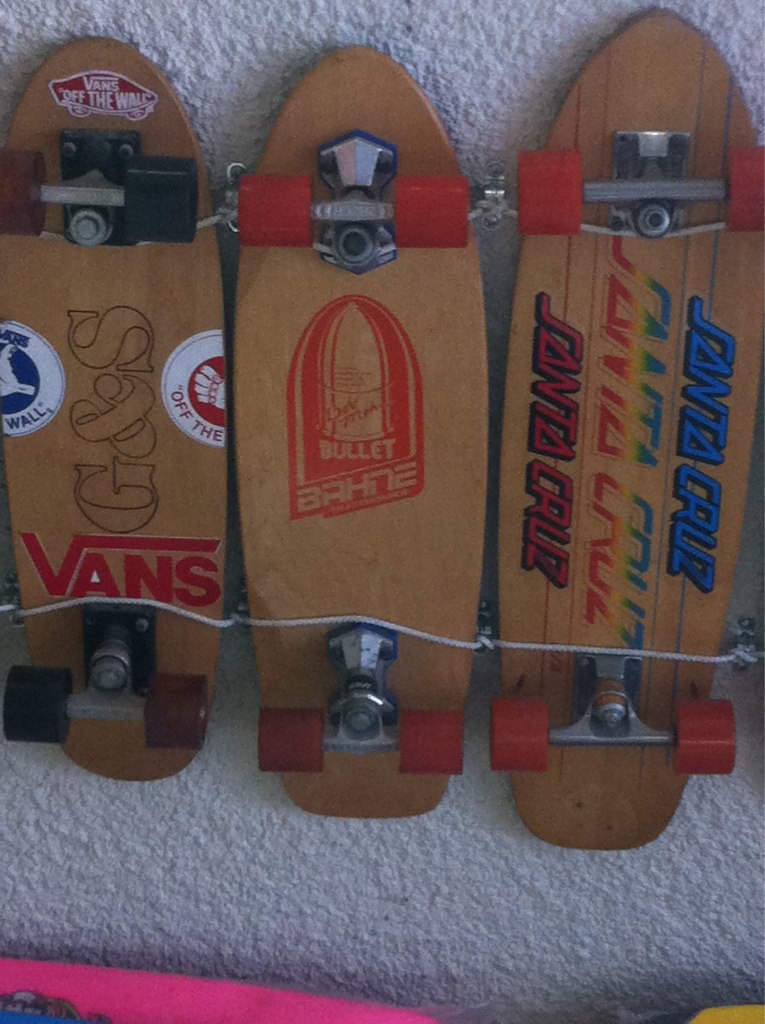The photograph features three vintage-looking wooden skateboards, laid out side by side, and displayed with their backs facing up. They are mounted on a concrete wall using wire mounts. These classic flat skateboards differ from modern designs and showcase distinctive logos. The first skateboard sports the "Vans Off The Wall" logo alongside "GNS." The second features the "Bullet" logo and the word "Bahn" in red. The third skateboard, which has vibrant designs, displays the "Santa Cruz" logo in blue, rainbow, and red fonts. All the skateboards are made of light-colored wood and have metal components attaching the wheels. Notably, two of them have red wheels, while one has a combination of black and maroon wheels. Additionally, there are intriguing splashes of color, with a pink element visible at the bottom left corner and a yellow one on the right-hand side.